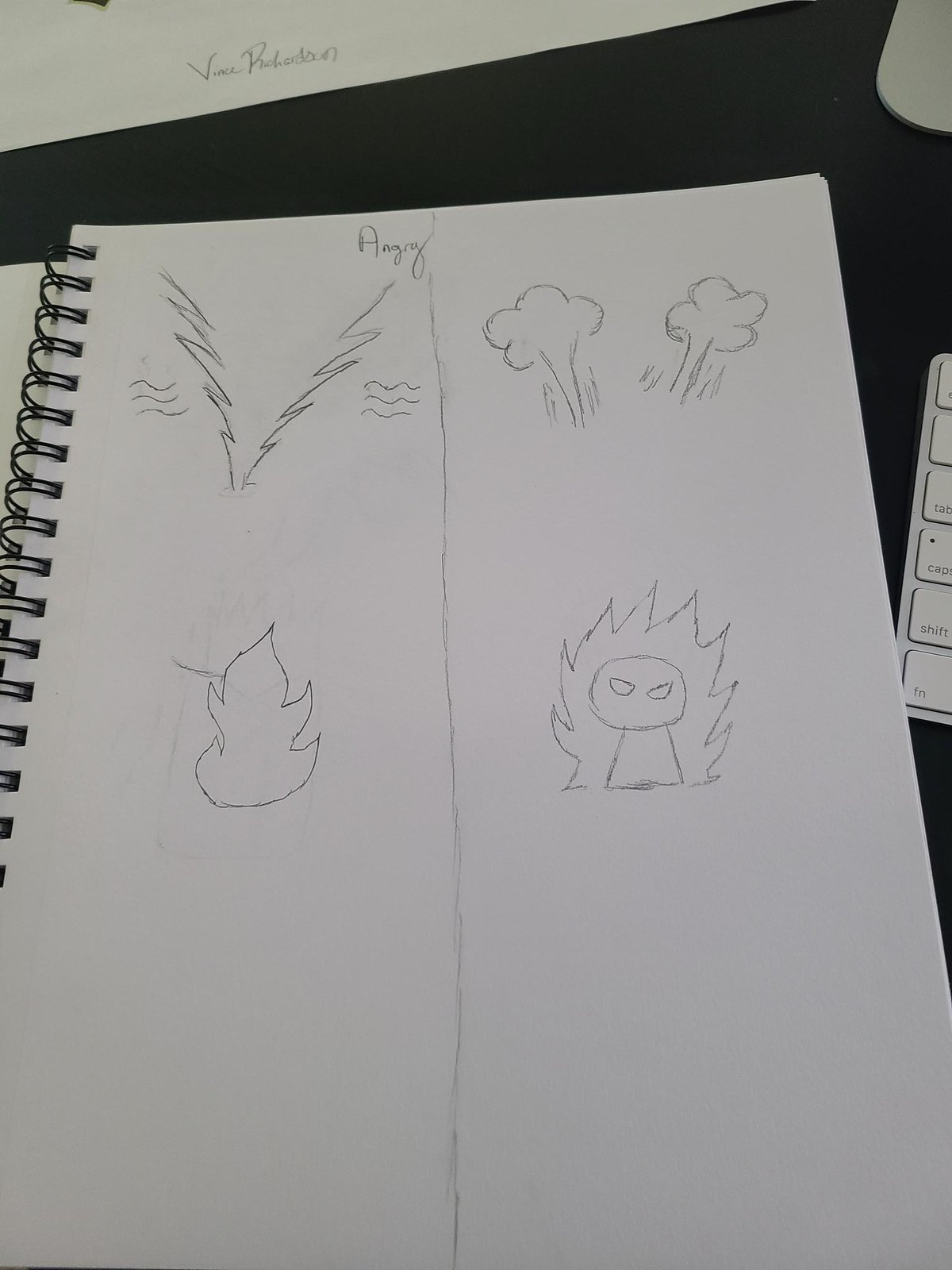A detailed photograph captures a plain sheet of white paper covered in various doodles and sketches, devoid of any lines. This page, likely a part of a sketchbook, rests on a dark-colored surface. On one side of the image, a series of black spirals are noticeable, suggesting the sketchbook's spiral binding. To the other side, there's a partial view of a white keyboard, and the top of the image reveals another sheet of white paper with some writing on it.

The main page features pencil inscriptions at the top and showcases four distinct doodles: two on each side. On the left side, abstract tree-like figures with wavy lines dominate the scene, with a flame illustrated below. On the right side, cloud or smoke-shaped objects occupy the upper portion, while a head and body figure with slanted, angry eyes, surrounded by flames, is prominently drawn below. The overall composition gives the feeling of an artist’s spontaneous and creative exploration.